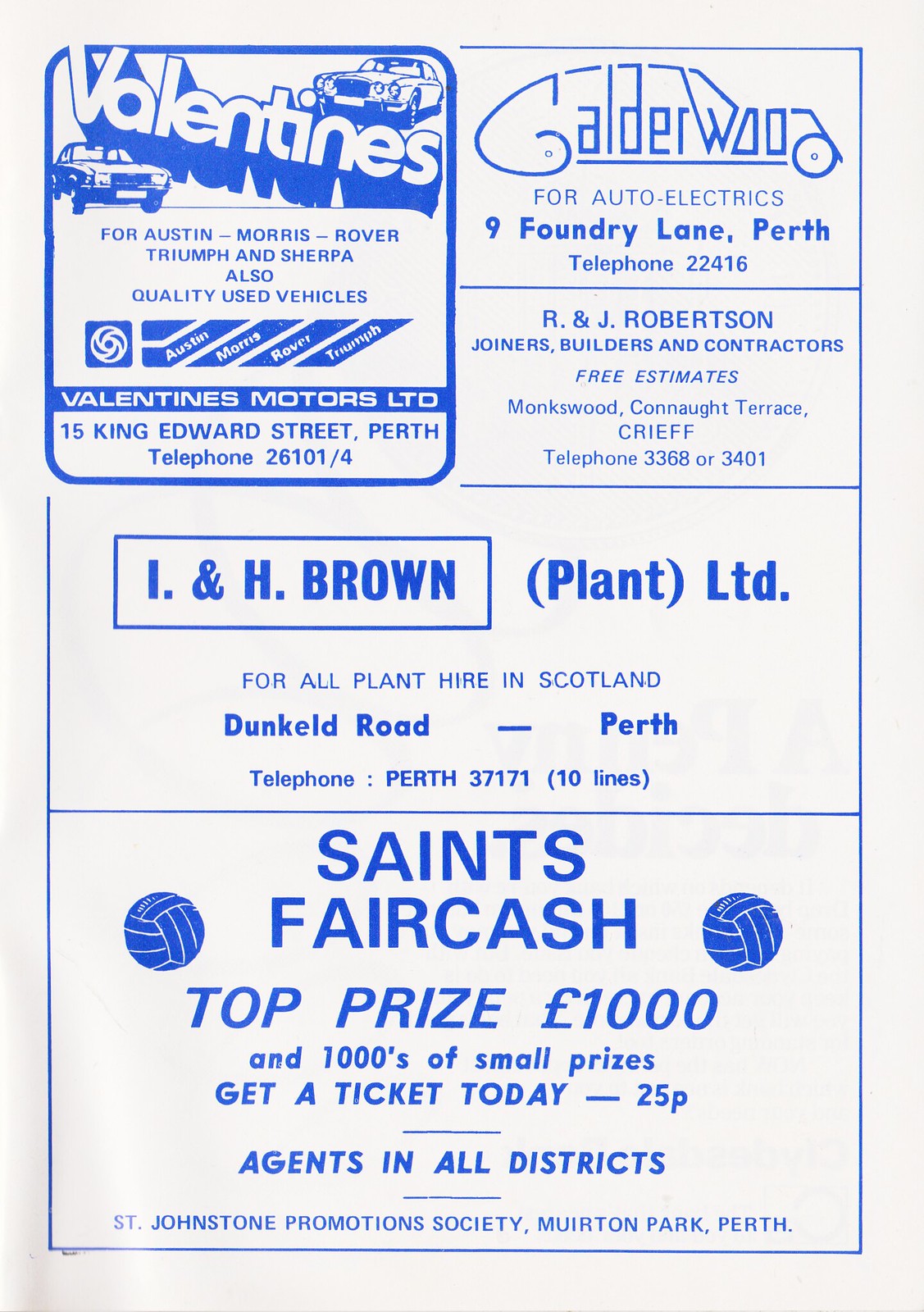This image features an aged advertisement page, likely from Perth, Australia, with a white background and distinguished by blue text and logos. The advertisement is divided into distinct sections, each bordered by blue lines.

- **Upper Left:** A promotion for Valentine's Motors, showcasing images of cars and providing an address and phone number.
- **Upper Right:** An ad for Calderwood Auto Electronics, also including an address, phone number, and the promise of free estimates. Nearby is an ad for R&J Robertson Builders and Contractors.
- **Middle Row:** An advertisement highlighting INH Brown Plant Ltd, a company specializing in plant hire services across Scotland, along with its specific contact information located on Duncan Road, Perth.
- **Bottom Section:** Details for "Saints Fair Cash," mentioning a top prize of £1,000 and numerous small prizes, encouraging ticket purchases at 25p each. It notes agents available in all districts, organized by the St. John's Stone Promotion Society, with a specific location at Mureton Park, Perth. This section is visually marked by two volleyball images.

Throughout the page, the blue text varies in size and style, giving each company's ad a unique presence while maintaining a cohesive look.